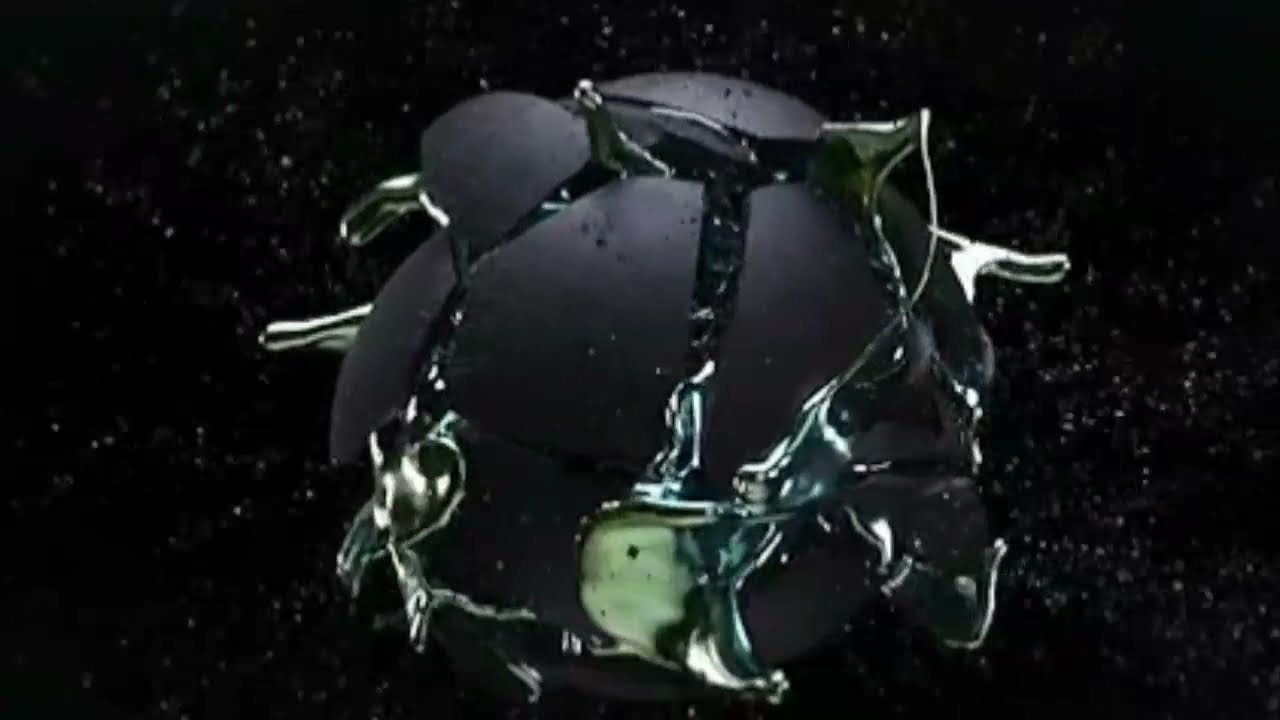The image depicts a highly detailed and artistic design that features a central black ball, situated against a pitch-black background peppered with white specks that resemble either stars in space or particles suspended in water. The ball appears shattered, with cracks spreading across its surface, exposing its inner contents. Emanating from the cracks is a variety of substances, including a silver liquid that flows out through the fractures and a green, gooey jelly-like material with off-white edges. The scattered bits and sparkles in the background create an impression of dynamic disintegration, enhancing the visual effect of the ball breaking apart. The overall color palette includes shades of black, gray, white, silver, blue, and green, contributing to the image’s striking and intricate composition.